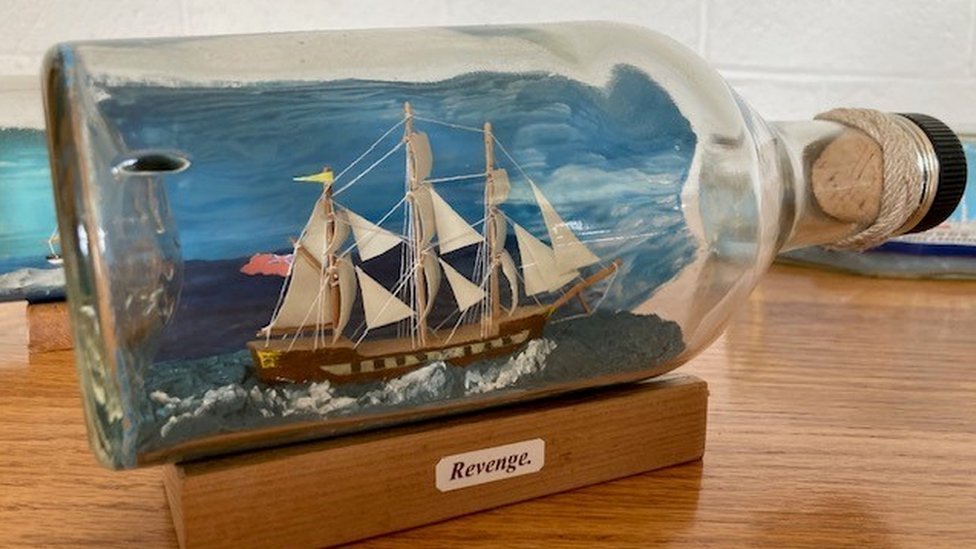This detailed photograph showcases a finely crafted ship-in-a-bottle display. The bottle, positioned on its side, features a black plastic cap secured with twine around the neck and a cork stopper. Inside the bottle, a meticulously constructed model ship appears to be sailing through an ocean, accentuated by a painted blue backdrop and choppy white-capped waves. The ship itself is a pirate-like vessel with a dark brown hull and a white deck, outfitted with three wooden masts adorned with multiple white sails, suggesting it is in full sail. The bottle is elegantly mounted on a wooden stand, which bears a silver tag inscribed with "REVENGE," likely the name of the ship. This entire setup is placed on a wood grain brown table, enhancing the nautical theme of the display.